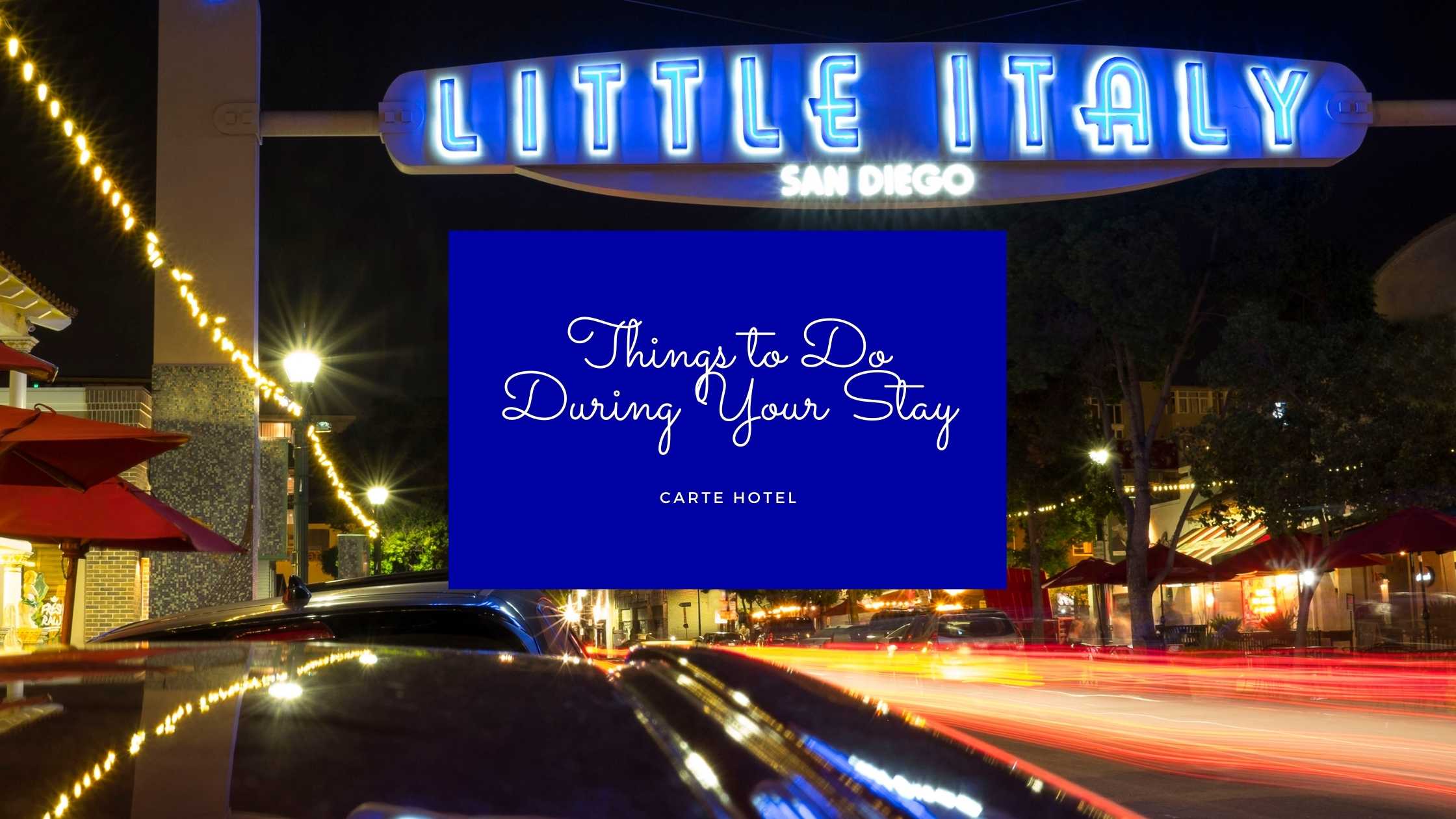This advertising image for Cartier Hotel captures the vibrant nightlife of Little Italy in San Diego. The photograph, taken from above a parked car on the left side of a bustling multi-lane street, features a large, illuminated signboard that stretches across the thoroughfare. The signboard, supported by two pillars, glows with blue and white neon lights and reads "Little Italy, San Diego." The street is flanked by well-lit restaurants and businesses, adorned with string lights and festive decor. There is a noticeable motion blur with red and white light streaks, suggesting the rapid movement of cars. Superimposed over the photograph is a blue rectangular box in the center with white cursive font that reads, "things to do during your stay. Cartier Hotel."